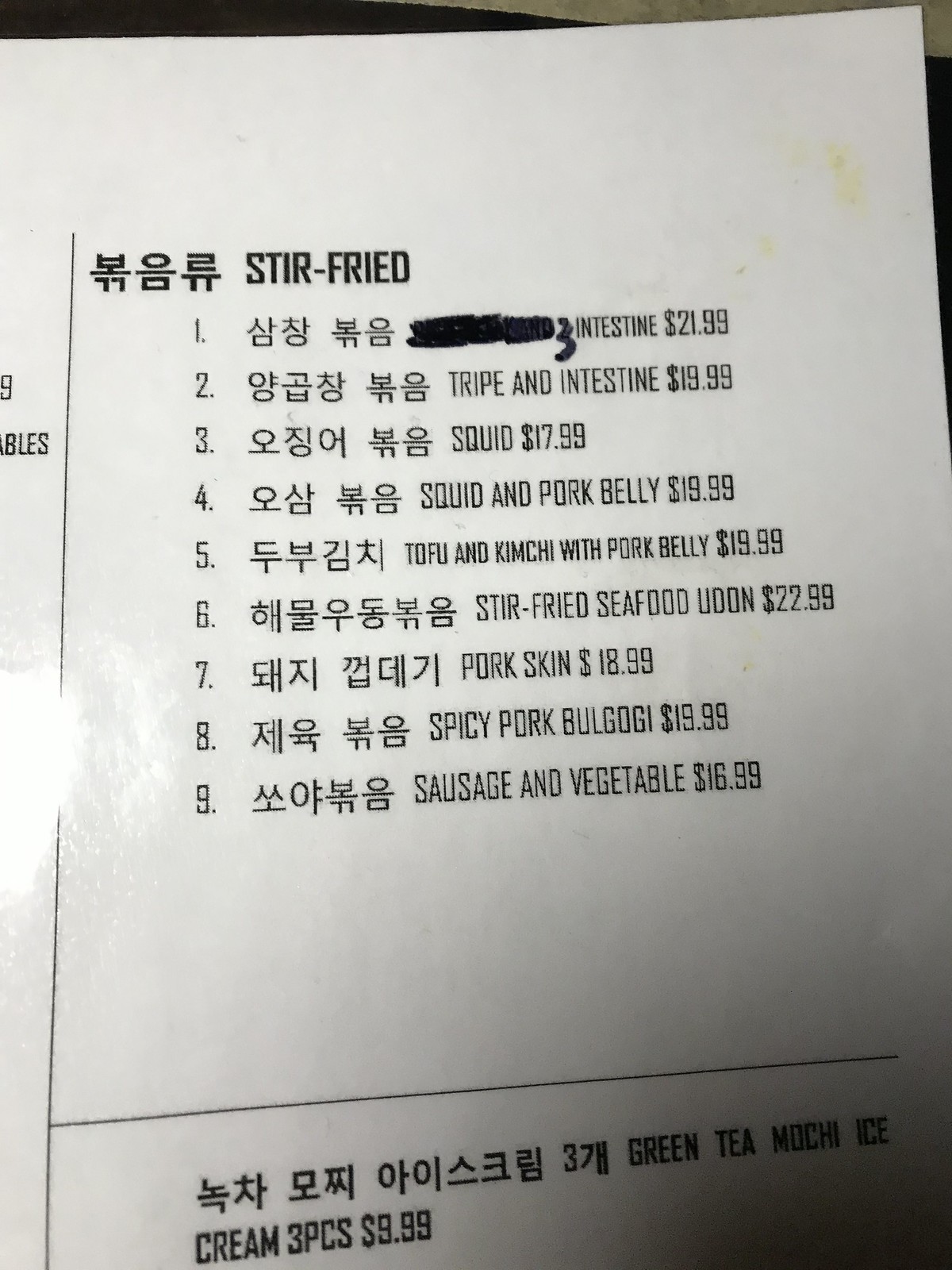This image captures a minimalistic menu presented on a white, almost laminated piece of paper. An illuminating flash is visible on the left side. The sparse layout is interrupted by some smudged, yellow stains on the top right. The menu features "STIR FRIED" written in bold black capital letters, flanked by Asian characters. Below, a detailed list of dishes numbered one through nine is provided, with each entry accompanied by Asian script and an English translation:

1. Stir-Fried Three Intestines - $21.99
2. Stir-Fried Tripe Intestines - $19.99
3. Stir-Fried Squid - $17.99
4. Stir-Fried Squid and Pork Belly - $19.99
5. Tofu and Kimchi with Pork Belly - $19.99
6. Stir-Fried Seafood Udon - $22.99
7. Stir-Fried Pork Skin - $18.99
8. Spicy Pork Bologna - $19.99
9. Sausage and Vegetables - $16.99

Beneath these items, separated by a line, additional Asian characters are visible. The final item on the menu is Green Tea Mochi Ice Cream (three pieces) priced at $3.99.